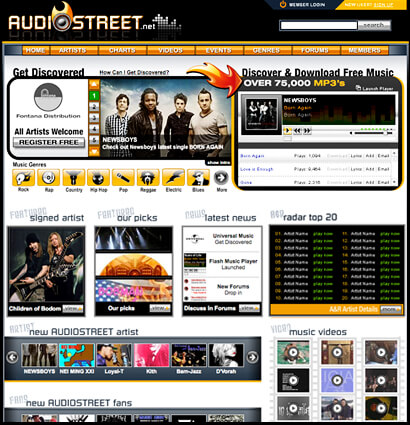This image is a detailed screenshot from the website AudioStreet.net. At the top, a black banner stretches across the page. Positioned on the left side of the banner is the AudioStreet logo, featuring the word "AudioStreet" in a bold, large yellow font. Notably, the "O" in "AudioStreet" is stylized to resemble a speaker engulfed in flames. Following this is ".net" in a smaller white font, accompanied by a series of squares.

On the top right side of the banner, there is a small "Login" button. Beneath this button is a yellow bar, which is difficult to read but likely contains a button or text link. Directly under the yellow bar is a text box for search functionality, accompanied by a sleek, silver search button.

Below the black banner, an orange navigation bar showcases various links to different pages within the site. These links include "Home," "Artists," "Charts," "Videos," "Events," "Genres," "Forums," and "Members," all displayed in an orange color with white font.

The main content area of the page features a large photograph of a band consisting of four members. Overlaying this image is a caption that reads, "Newsboys, check out Newsboys' latest single." 

To the top right of the central image, there is an illustration resembling an MP3 player app, complete with a playlist of songs displayed. The rest of the page maintains a clean, white background that emphasizes the colorful elements and content sections of the site.